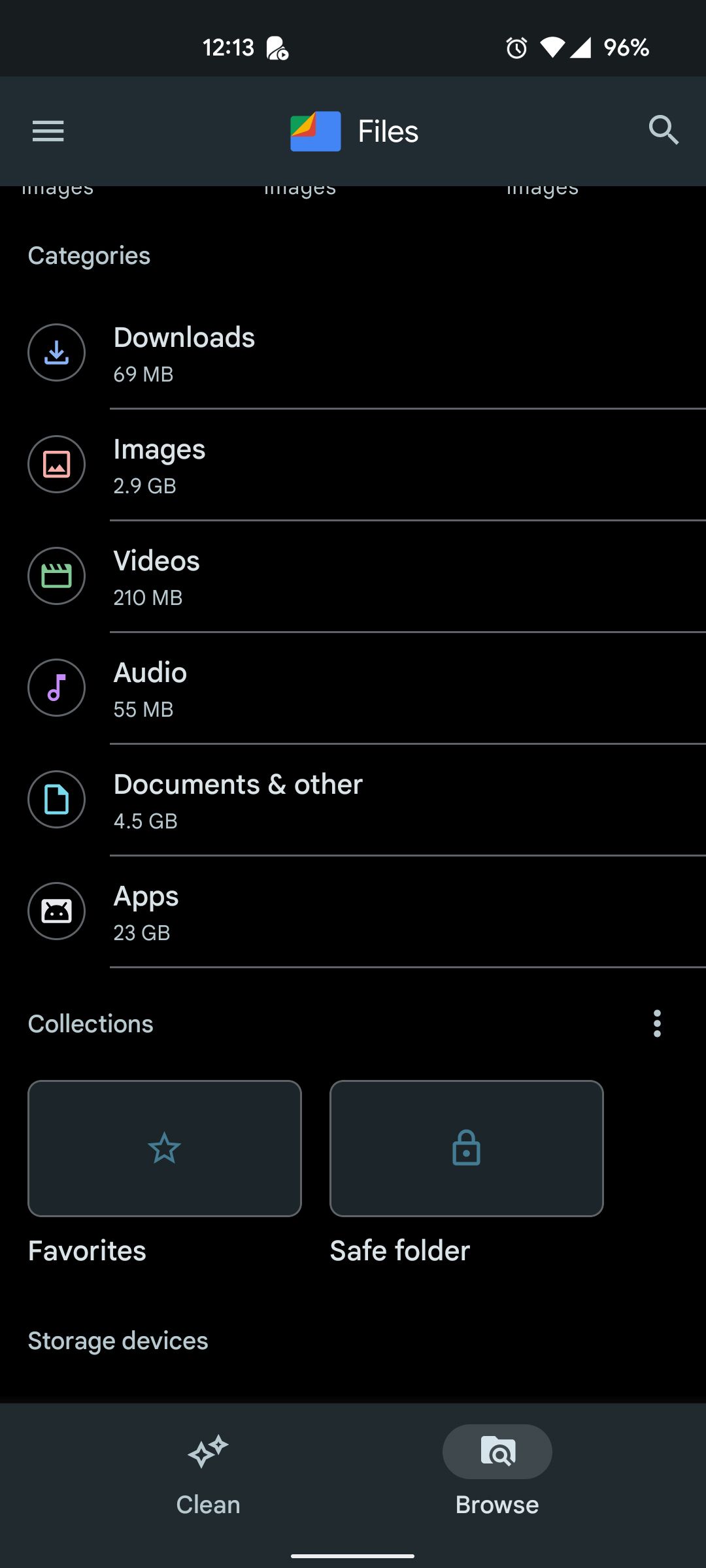This is a detailed screenshot from a cell phone displaying the files directory interface. The background is predominantly black, providing a high-contrast setting for the various icons and text. The top section of the screen features white text, including the current time displayed as 12:13. In the upper right-hand corner, several status icons are visible: an alarm clock, a Wi-Fi symbol, a cell phone signal indicator, and a battery level showing 96% charged.

A gray banner stretches across the top of the page, centrally highlighted by a colorful square logo emblazoned in blue, yellow, red, and green, next to which the word "Files" is prominently displayed. Below this gray banner, the main content area also has a black background with light gray text detailing different file categories and their respective storage sizes: "Categories", "Downloads 69 MB", "Images 2.9 GB", "Videos 210 MB", "Audio 55 MB", "Documents and other 4.5 GB", and "Apps 23 GB".

At the bottom of the screen, aligned horizontally under the word "Collections," are two rectangular buttons. The button on the left showcases a star icon at its center, while the button on the right features a lock icon. Below these buttons are the labels "Favorites" and "Safe folder," respectively, denoting their functionalities.